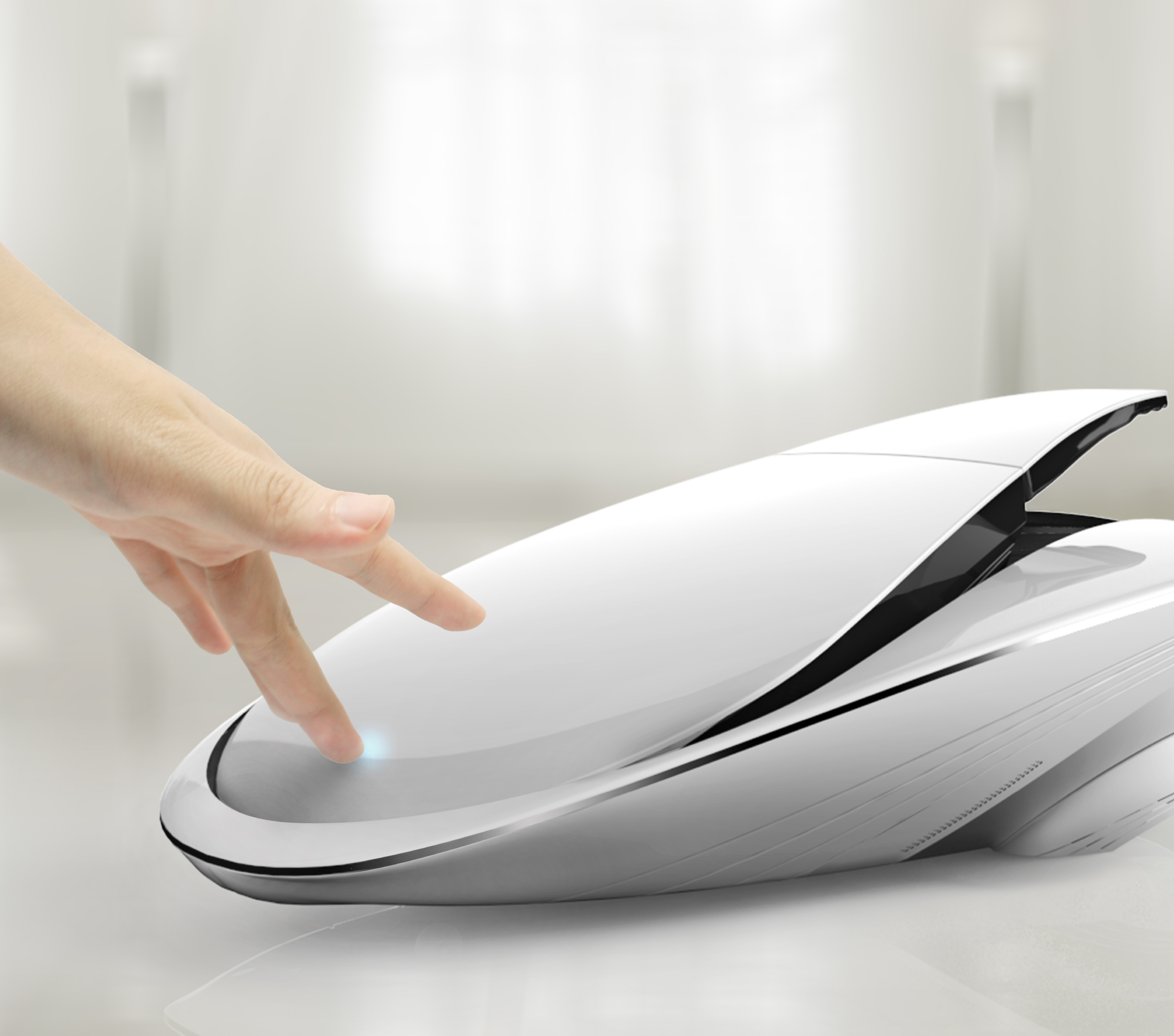This full-color, indoor photograph, taken under artificial light, centers on a sleek, teardrop-shaped household device made of shiny white plastic with a silver trim. The image is square and set against a plain background, showing a contrasting countertop beneath the main object. A Caucasian hand, gender indeterminate, enters from the left-center, pressing on the glowing blue touch-sensitive front of the device, which tapers downwards and features a curvy body. The fingers push inward, causing a back panel with a white flap to open, revealing a black interior. In the top-center is a softly lit rectangular form resembling a window or screen. The device appears to have a modern, high-tech style, hinting at a new type of machine, possibly related to home cleaning, given its resemblance to a vacuum cleaner canister and the presence of small round wheels on the far right base. The dominant colors in the image are white, black, gray, beige, and a hint of glowing blue light.